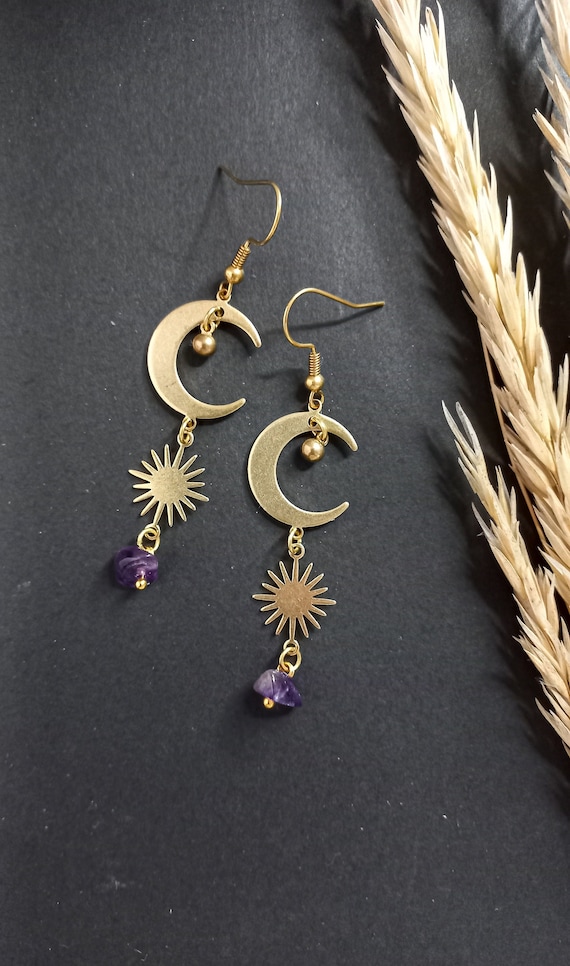This is a close-up photo of a pair of exquisite gold dangle earrings resting on a black background, possibly felt, that gives the backdrop a rich texture. Along the right border of the image, there is a sprig of dried wheat or rice, adding a rustic touch with its golden-ivory hues. The earrings feature elegant fish hook wires, each adorned with a tiny spring and a gold bead. Below the hooks, a series of elements create a cascading effect: a stylized crescent moon with a small gold bead nestled inside the curve, a delicate chain extending down to a gold starburst, and finally, a rough amethyst bead that adds a pop of rich purple at the bottom. Both earrings are designed symmetrically, with the left one slightly raised compared to the right. The composition, likely arranged for advertisement, highlights the intricate details and elegant craftsmanship of the earrings.